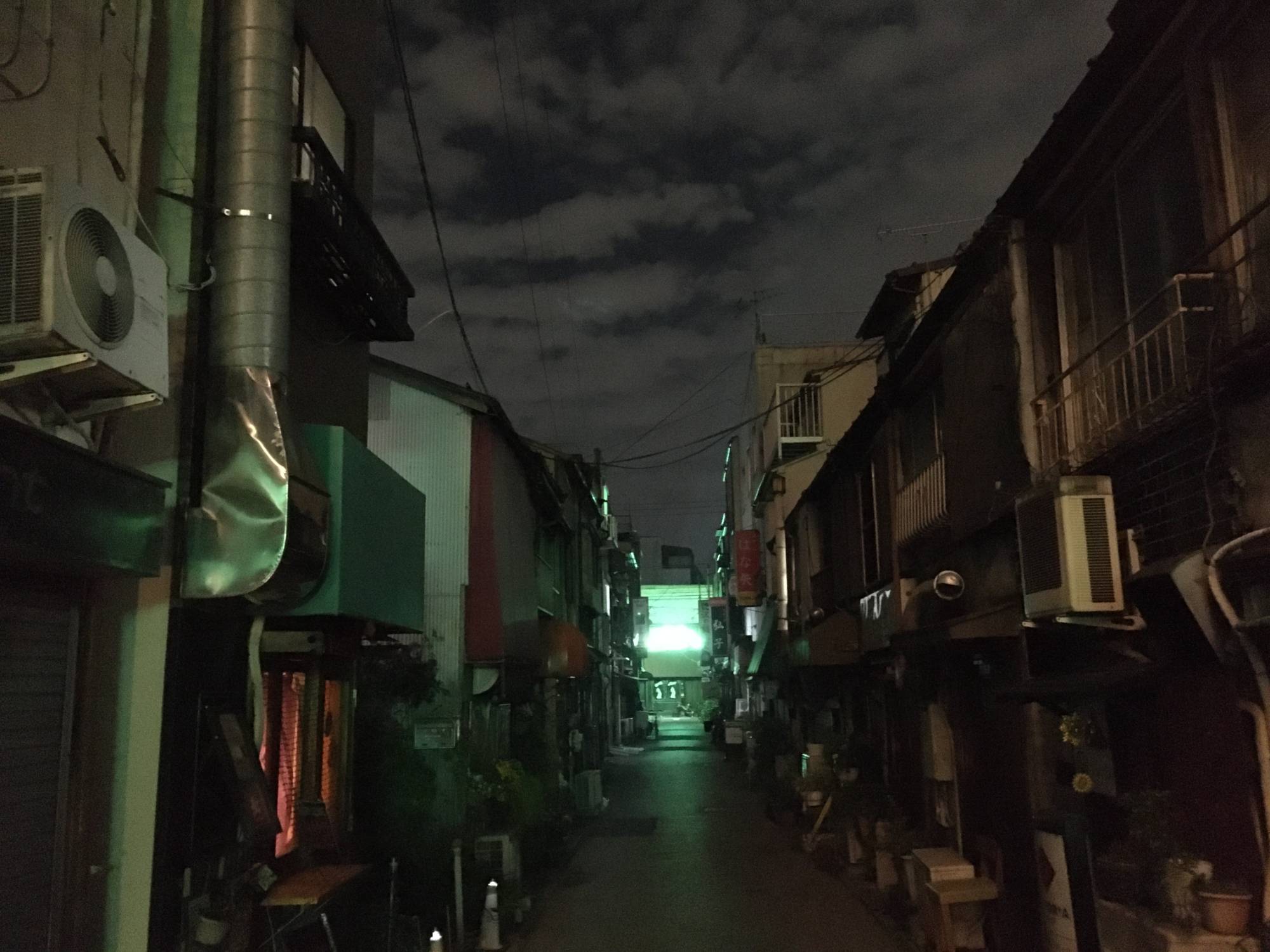A square, full-color night photograph taken outdoors in an Asian town. The scene is illuminated with artificial lighting, revealing an overcast, gray sky that emphasizes the nighttime setting. At the center of the image is a striking, bright green neon sign, which stands out as the primary light source in the scene. The view is from street level and captures a narrow alleyway formed by close-set apartment buildings on either side, appearing to close in slightly. The alleyway leads to a mysterious wall, adding to the eerie atmosphere. The architecture is predominantly dark and muted, with colors including mint green, reddish hues, grays, whites, and blacks. Notably, there are signs with Asian characters, affirming the setting, but no people are visible, enhancing the isolated and creepy ambiance.